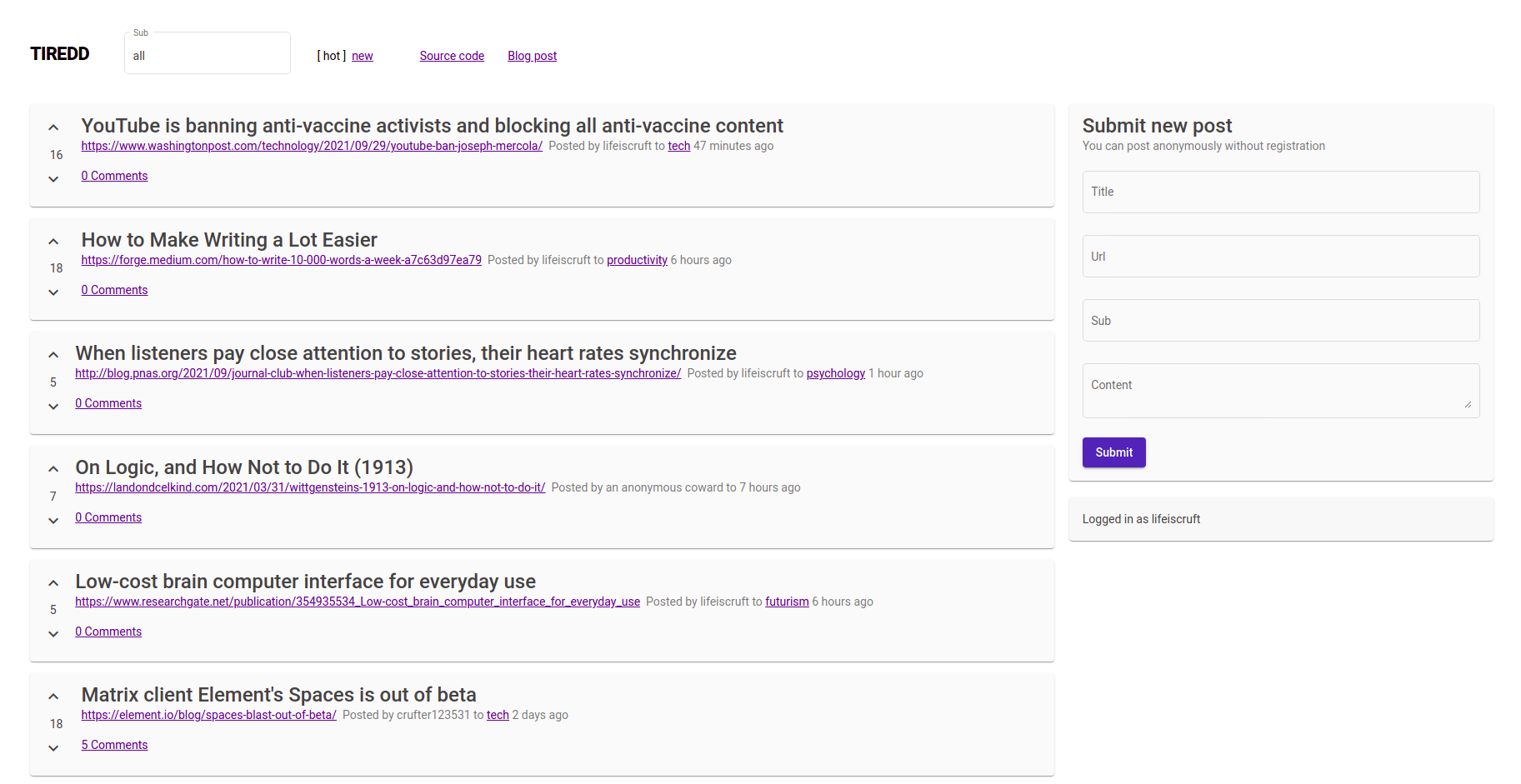In the image, there is a white background with the title "Tired-O" displayed prominently in black print at the top. Below the title is a small blue box. The image also features sections highlighted in light purple and numerous light purple boxes.

On the left side of the image, there are light purple boxes each containing small up and down arrows with numbers between them. These boxes include black print text that says "YouTube is banning anti-vaccine activists and blocking all anti-vaccine content." Underneath this text, there is a purple line with purple writing.

Further down, additional content in purple writing includes topics such as "How to make writing a lot easier," "When listeners pay close attention to stories their heart rates synchronize," "On logic and how not to do it," "1913 low-code brain-computer interface for everyday use," and "Matrix client Element Spaces is out of beta."

On the right side of the image, there is a light purple box labeled "Submit new post." This box includes fields for a title (appearing as "UVI"), a subtitle, and an option. There is also a purple button with white text that says "Submit," along with a statement "I agree to their terms."

Overall, the composition combines various sections and topics with a predominant use of purple and white colors, alongside black print for key information.